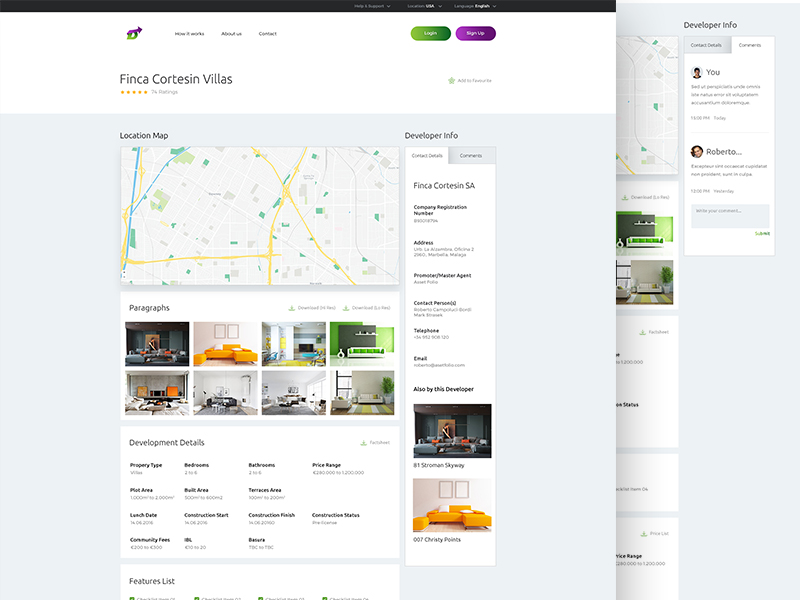This is a detailed screenshot of a real estate website showcasing information about a property. The layout features two overlapping versions of the webpage, with the primary version fully visible on the left and the secondary, slightly darkened version partially visible behind it to the right. 

The header has a white background. In the top left corner, there's a logo featuring a purple arrow pointing upwards and to the right, with a green "D" underneath. To the right of the logo are three gray text areas labeled "How it works," "About us," and "Contact." Further to the right, there's a green, pill-shaped button with a slight gradient and white text reading "Log in," followed by a purple button with white text saying "Sign up."

Beneath the header, the title "Finca Cortesin Villas" is prominently displayed in large gray text. Directly below the title, a gold star rating is shown, with "74 ratings" indicated in light gray text to the right.

The main body of the webpage features a light bluish-gray background. At the top left, the text "Location map" appears in gray, followed by a rectangular map beneath it. The map displays a network of yellow and white roads. A central feature of the map is a yellow road intersection forming an "X" towards the center-right of the image. One leg of this "X" extends downward and to the left before making a 90-degree turn upward. The white roads on the map create grids set at various angles across the area.